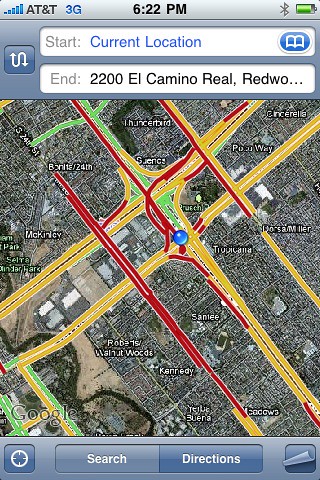The image displays the screen of a smartphone with a silver-gray perimeter. In the upper left corner of the screen, AT&T is indicated as the service provider alongside a barcode symbol, showing a full signal strength of five bars. The phone operates on a 3G network. On the upper right corner, the battery level is nearly full, and the time reads 6:22 p.m. 

The current location is highlighted as 2200 El Camino Real, identified as being in Redwood. The map showcases major intersections, likely multi-lane highways, suggesting a highly urbanized and congested area. Prominent street names visible include El Camino and Kennedy. At the bottom of the screen, navigation options such as 'Search' and 'Directions' are displayed. There is also a button labeled 'Page' and another in the lower left corner for movement or navigation directions, though the associated text is unclear. 'Tropicana' and other various names appear on the map, contributing to the depiction of a bustling urban environment with numerous houses and small cross streets visible in the background.